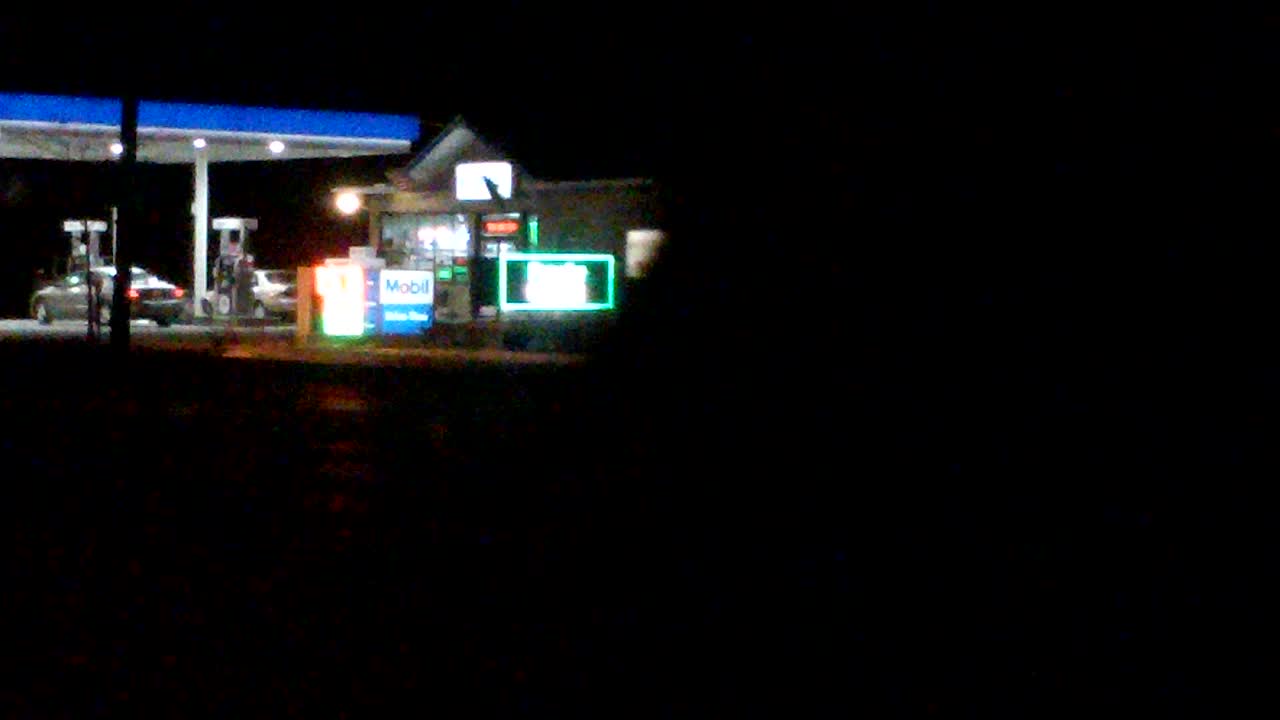This evocative nighttime photograph captures a gas station bathed in a pool of artificial light amidst an otherwise dark and shadowy environment. The focal point is the bright Mobil sign, each letter of "M-O-B-I-L" vividly standing out against the night sky. Below the sign, the gas station building is partially visible and illuminated, giving a sense of activity and presence. The canopy, supported by sleek columns, shelters the gas pumps beneath it. Two sedans are parked at the pumps; one car's brake lights glow a vivid red, suggesting it has just arrived. Nearby, several other illuminated signs hint at additional services but remain indistinct due to blur, adding a sense of mystery. The station's windows throw out soft, diffused light, offering a glimpse of the interior but retaining an air of intrigue due to the distance and slight blur. The combination of sharp and soft elements creates a cinematic atmosphere, drawing the viewer into this nocturnal scene.